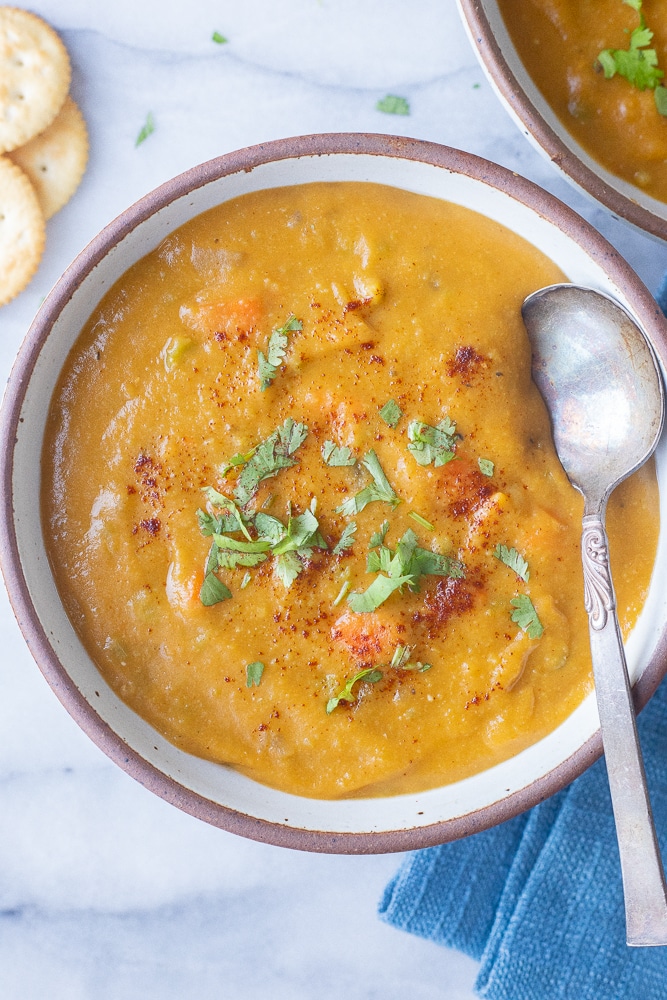The image showcases a richly colored bowl of thick, orange-yellow soup, garnished with green chives and a sprinkling of red powder. Pieces of carrots are visible beneath the surface, hinting at a hearty mixture. The soup is housed in a white bowl adorned with a red rim, and a spoon is partially submerged within, indicating readiness for eating. To the upper left, three circular crackers, reminiscent of Ritz, lay stacked, adding an inviting crunch to the ensemble. The top right reveals a second, similar bowl, possibly containing a darker variation of the same soup due to its placement in the background. Both bowls rest on a blue and white surface, complemented by a neatly folded blue napkin at the bottom right.